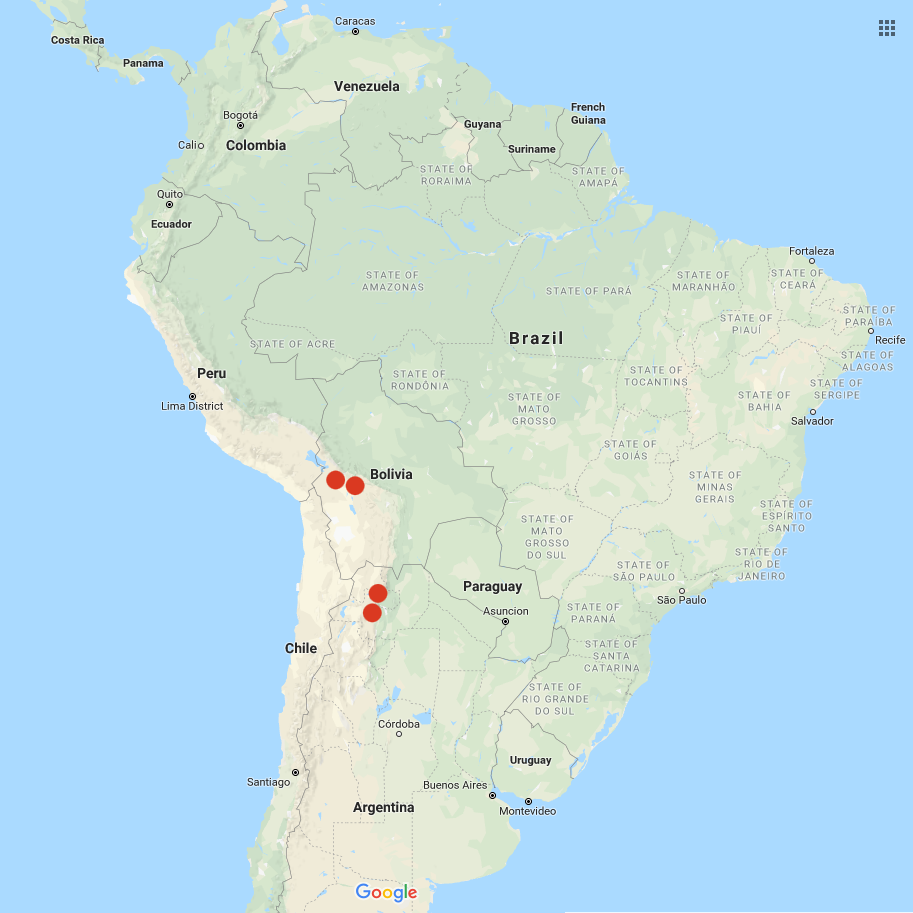The image depicts a detailed map of South America, highlighting the main countries: Venezuela, Colombia, Brazil, Bolivia, Paraguay, Chile, Argentina, and Uruguay. Notable features include two distinct red dots positioned in Bolivia and two similarly marked red dots in Argentina. The continent is surrounded by blue water, emphasizing the geographical boundaries.